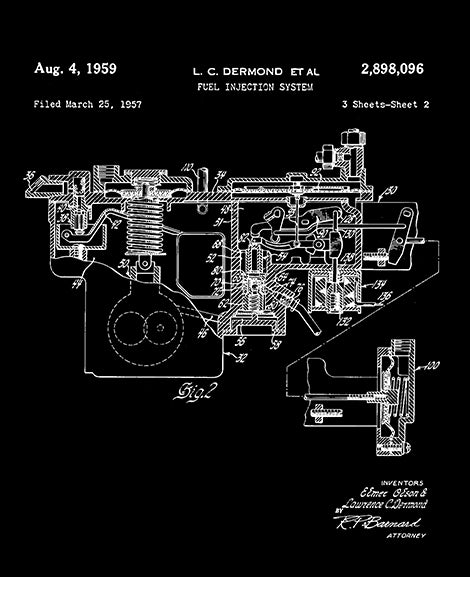The image depicts a patent paper for a fuel injection system designed by L.C. Dermond et al., against a stark black background. The top of the image features white text stating "August 4, 1959, filed March 25, 1957," followed by "L.C. Dermond et al. Fuel Injection System 2898-096, three sheets, sheet two." Below this text, there is a detailed white schematic of an engine's inner workings. Various components are annotated with numbered arrows, such as an arrow labeled "134," another marked "46," and a section reading "100." At the bottom, the inventors' names and the responsible attorney's details are noted.